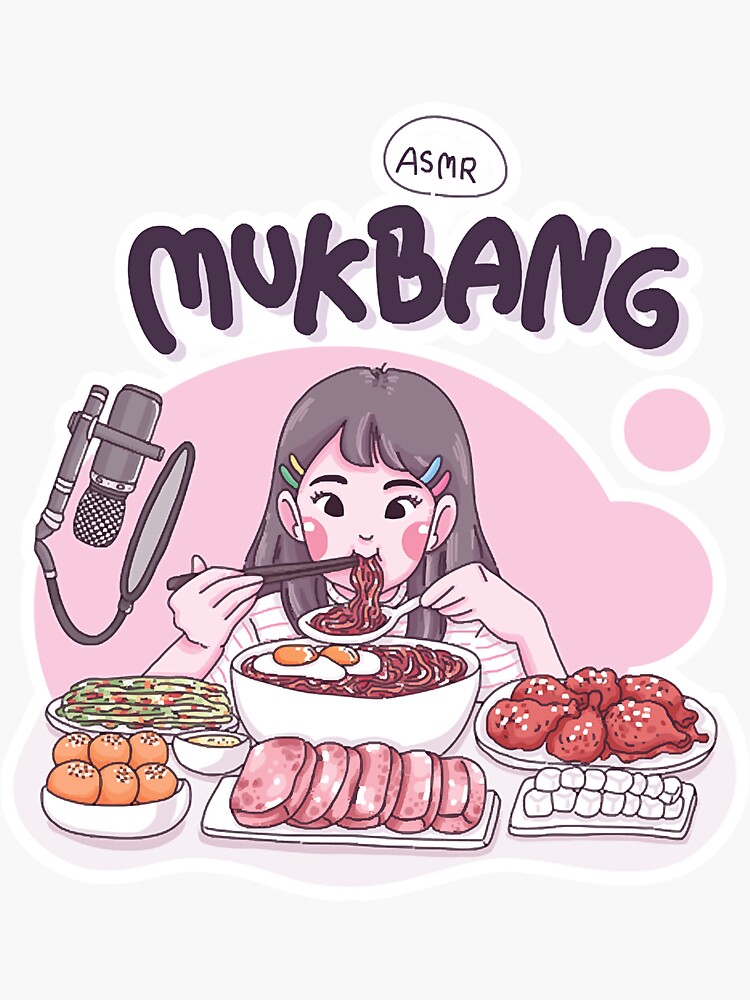The vertical, borderless cartoon-style image appears to be an advertisement with the title “ASMR Mukbang” prominently displayed in a purple bubble font across the top, with "ASMR" encapsulated within a speech bubble above it. Below the title, a girl with vibrant purple hair adorned with colorful barrettes (blue and pink on her right, yellow and green on her left) is featured eating noodles with purple chopsticks. She has pink cheeks and is wearing a white shirt with purple stripes. The background behind her comprises a large pink cloud-like shape with a smaller pink circle to the right.

In front of the girl, there is a variety of food meticulously presented: a white bowl filled with red noodles topped with two yellow and white eggs, a long white plate with pink and white Spam-like slices, yellow and red corn on a white plate, and another white bowl containing something yellow. Additionally, there is a dish with what looks like brownish-orange hard-boiled eggs speckled with brown, a plate of green and red kimchi-like items, a plate of brown chicken wings with white garnishes, and a plate of white marshmallow-like items. To the left side of the image, there's a purple and white microphone with a pop filter positioned in front of it.